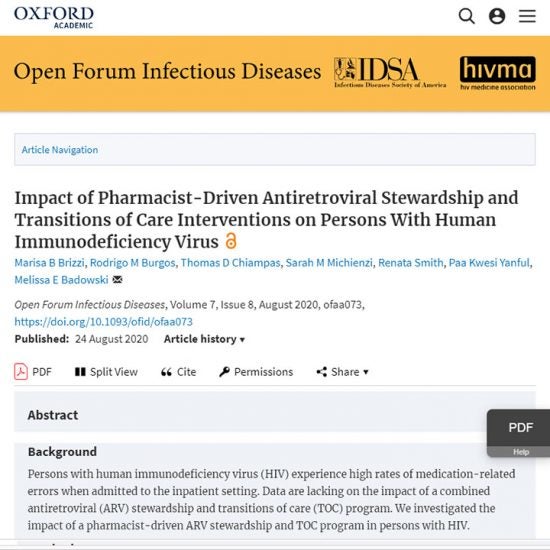This is a detailed screenshot of a website from Oxford Academic. At the very top, a white bar displays the text "Oxford Academic" in black font. Located on the right side of this bar are three icons: a magnifying glass, a black circle with a white human silhouette, and three vertically aligned black lines placed horizontally. 

Beneath this, there's an orange banner featuring the text "Open Forum Infectious Diseases IDSA," with "HFMA" written in orange and enclosed in a black rectangle. Below the orange banner, a blue rectangle contains the phrase "Article Navigation" in blue font.

The article's headline, written in bold black font, reads "Impact of Pharmacist-Driven Anti-Retroviral Stewardship and Transitions of Care Interventions on Persons with Human Immunodeficiency Virus." An orange open padlock symbol appears next to the headline. The authors of the article are listed in blue font: Marissa B. Berrizzi, Rodrigo M. Burgos, and Thomas D. Chiampas.